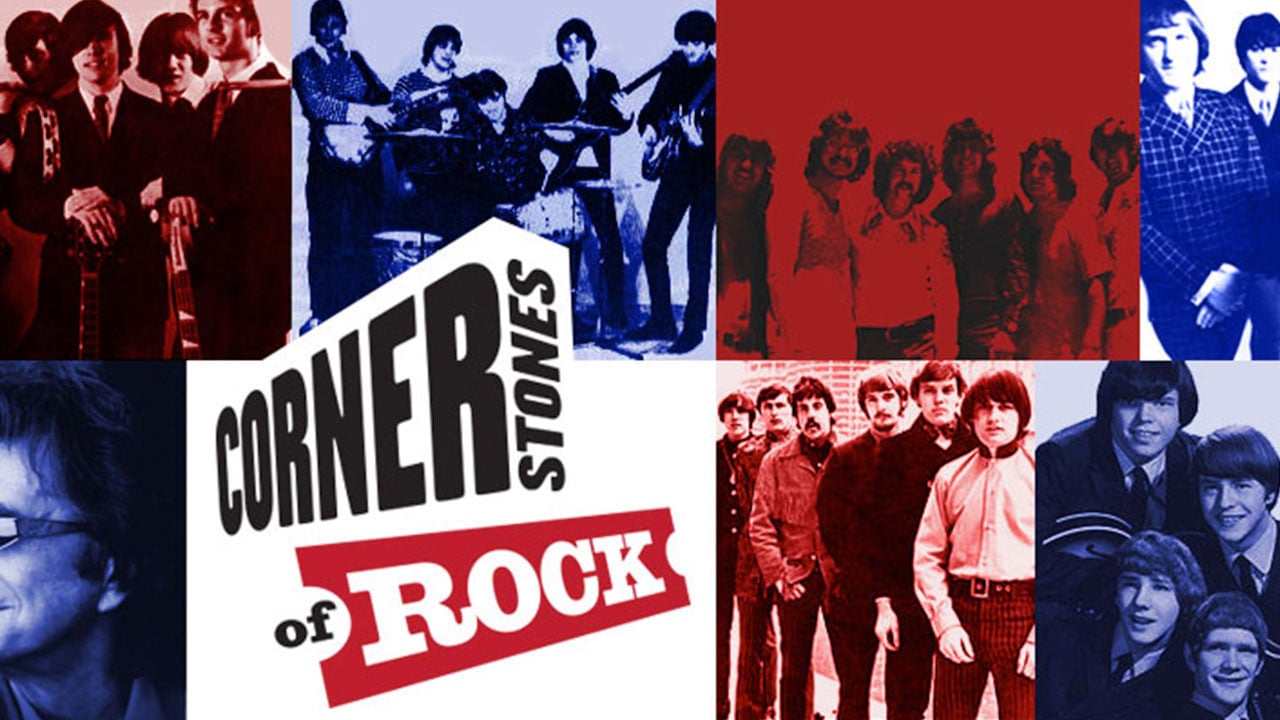This image is a detailed collage reminiscent of something you might find at the Rock and Roll Hall of Fame, presenting an assembly of iconic rock bands from the 50s, 60s, and 70s. The overall layout is in a landscape orientation, featuring seven black and white photographs tinted with various colors—light red, light blue, dark red, and pink. These photos capture promo shots of young men with long hair, some with facial hair, standing together, representative of the era's bands.

In the bottom left of the image, there's a white rectangular area with stylized text that reads "Cornerstones of Rock." This text design integrates the words "Corner" and "Stones" perpendicularly, forming a corner-like block. Below it, the word "Rock" appears in white letters against a red strip, designed to resemble a ticket. Notably, the collage includes recognizable figures such as Bob Dylan, positioned in a light blue tinted profile on the bottom left, and The Beatles and The Rolling Stones, identified among the other prominent bands. The design style blends photographic realism with graphic design elements and color filters, creating a timeless tribute to the foundational legends of rock music.